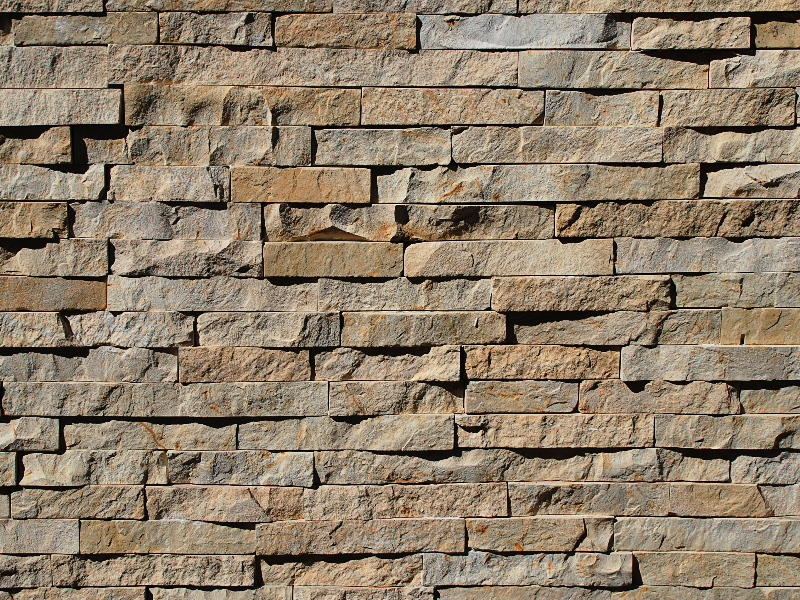This is a close-up photograph of a large stone wall constructed from granite slab bricks. The wall is tightly stacked with rectangular, uniformly thick bricks that have irregular, undulating front surfaces, making some stones protrude more than others. These bricks range in color from predominant grays to occasional sandstone and yellowish tones, giving the wall a varied but muted earth-like appearance. The well-lit setting enhances the contrast, casting stark shadows beneath the protrusions and emphasizing the texture and depth of the wall. There is no visible mortar between the bricks, suggesting a dry-stack construction method. The photograph is solely focused on this monotone, textured wall, offering no background elements or labels, making it somewhat monotonous and leaving its function—possibly as a retaining wall or part of a building facade—ambiguous.